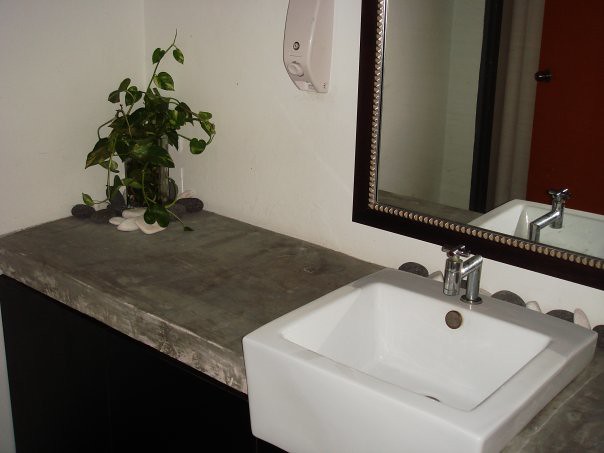This photograph captures the sophisticated interior of a public bathroom, viewed from a side angle that highlights the left-hand section. The room features a moderately-sized grayish countertop, meticulously blending varying shades of gray to create a granite-like, marbled appearance. Nestled in one corner of the countertop is a lush green plant, housed in a sleek, black vase, with its vibrant leaves cascading over the edges. Nearby, a few small white objects rest against the base of the plant, adding a subtle contrast.

Prominently situated on the countertop is a deep, square-shaped white basin sink, which extends forward, obscuring the edge of the gray countertop from view. The sink is complemented by a polished silver faucet. Above this setup, a rectangular mirror framed in dark brown adds an element of elegance. The frame features a decorative design, adorned with tiny gold circles arranged closely together, enhancing the mirror with a refined, ornate secondary border.